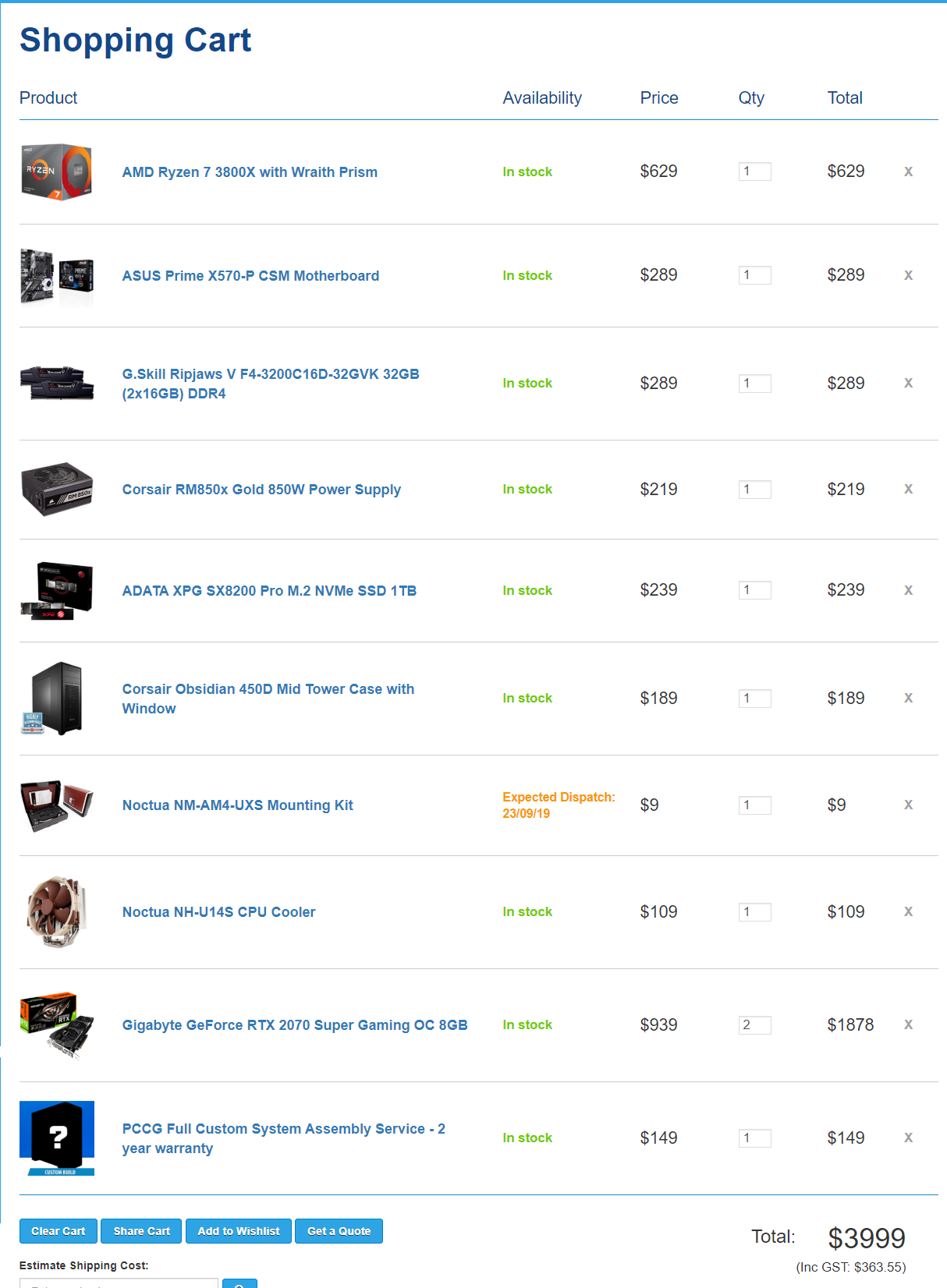The image features a detailed screenshot of an online shopping cart page from a website. The page is framed by a distinct thicker blue border at the top, a thinner border on the left side and bottom, while the right side remains borderless. At the top, it clearly states "Shopping Cart."

Beneath the header, there is a column titled "Product," showcasing a vertical list of product images. Each product is accompanied by its own picture and a full description written in blue text. Next to each product description is an "Availability" column indicating the stock status. Items that are available are marked in green, while one product, "Noculus," is highlighted in orange with an "Expected Dispatch" date of June 19, 2023.

Following the availability column, the page displays the price of each item, a column for the quantity, and the total price for each product. Notably, the total price for the "Noculus," which hasn't arrived yet, is marked as $0. The sum total of all the products in the cart is $3,999, alongside an included GST of $363.55.

At the bottom left corner, there are several action buttons labeled "Shopping Cart," "Show Cart," "Add to Wishlist," and "Get a Quote." The page also mentions an estimated shipping cost, but this information appears to be cut off, implying that it would typically be clickable for further details.